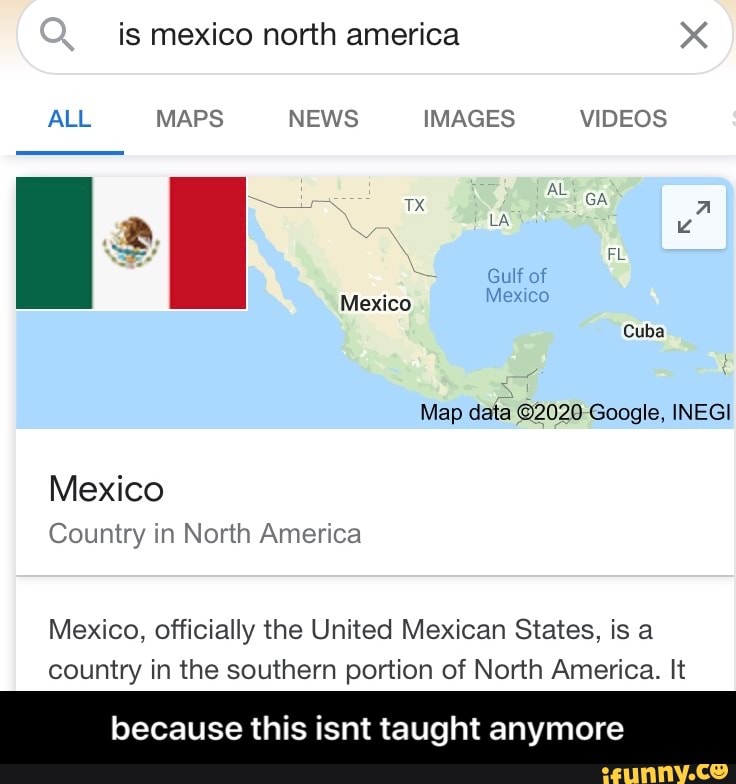A search results page displays information related to Mexico, North America. The search bar, located at the top, features a magnifying glass icon on the left and an "X" on the right. The navigation tabs below the search bar are labeled as 'Maps', 'News', 'Images', 'Videos', with 'All' highlighted and underlined in blue. 

The main page displays a map highlighting Mexico, along with neighboring regions such as Cuba, the Gulf of Mexico, Texas (TX), Louisiana (LA), Alabama (AL), Georgia (GA), and Florida (FL). Additionally, the page includes the Mexican flag, which is tri-colored green, white, and red.

At the bottom of the map, a copyright notice reads "Map data ©2020 Google, INEGI." There is also a brief description of Mexico, noting it as a country in the southern portion of North America, officially named the United Mexican States.

An overlay element features a black rectangle with white text stating, "because this isn't taught anymore." Below this, in yellow text, is the watermark "ifunny.co," where the ‘O’ is stylized as a smiling face.